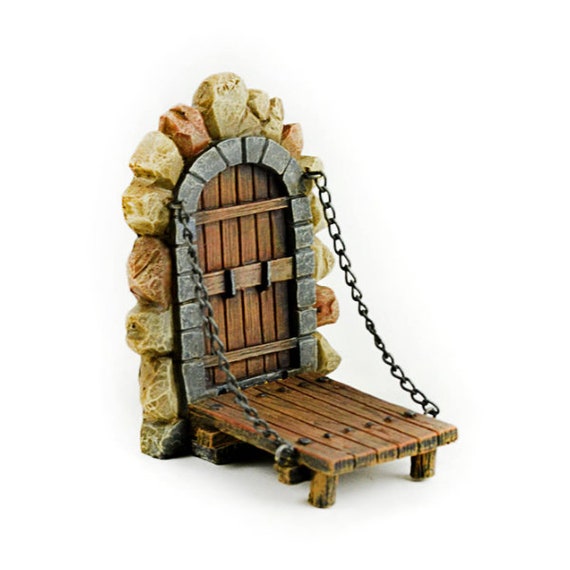The image depicts a detailed miniature model resembling a castle drawbridge and doorway. The door is a semi-circular, medium brown wood structure with vertical slats and three horizontal support bars. It is flanked by two heavy chains, which can be maneuvered to lift the drawbridge. Surrounding the door is intricate stonework featuring an arch of cut gray stones that seamlessly mimic the curve of the doorway. Encompassing this gray section are larger, natural-looking stones in shades of tan and rust. The drawbridge itself has wooden beams and is secured with large bolts, adding to the authentic castle-like appearance of the scene. The model appears to be made of resin and is reminiscent of a detailed display in a hobbyist collection.